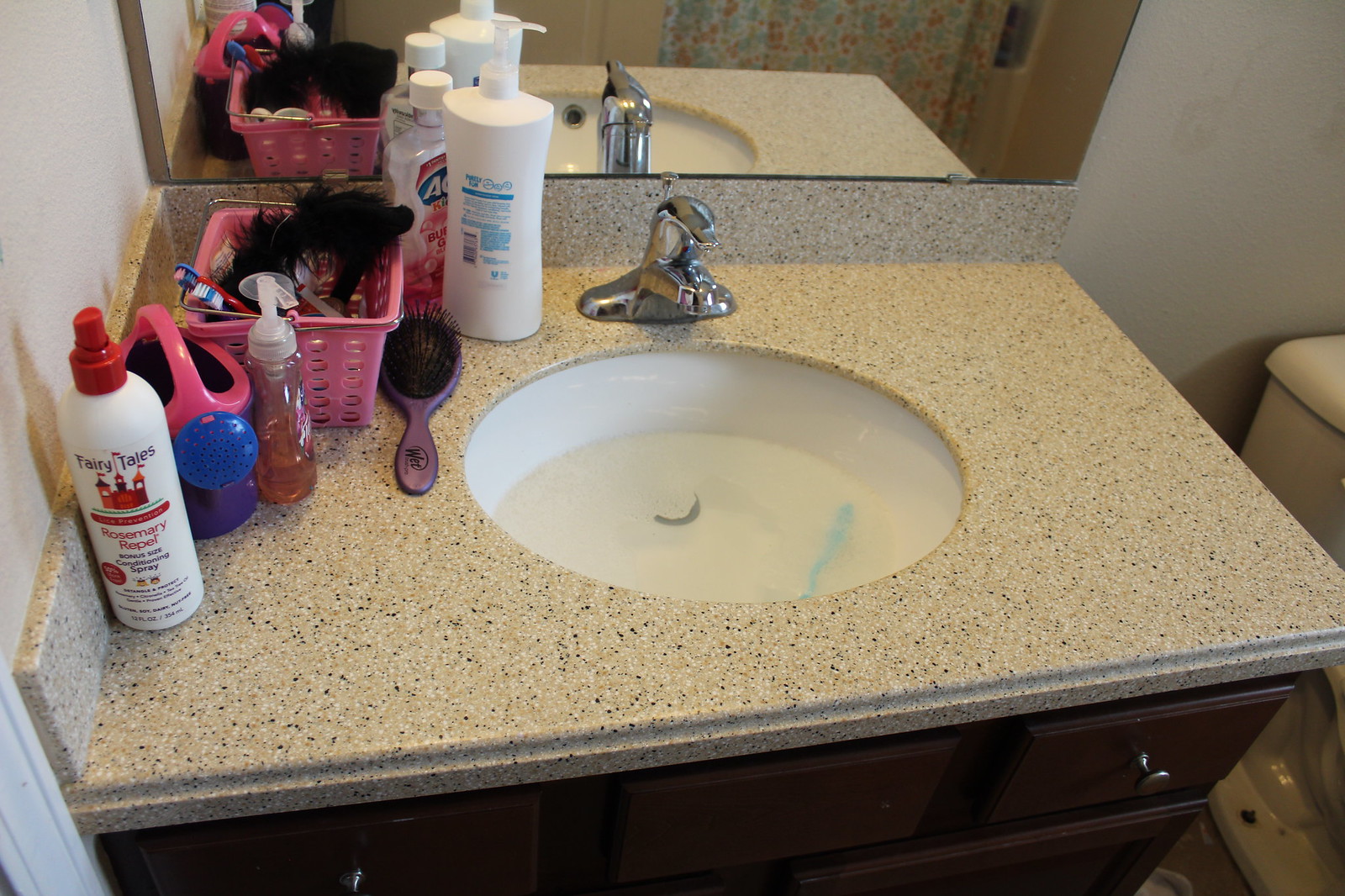This photograph, taken in landscape mode, captures a corner view of a residential bathroom focusing on a sink and vanity unit. The pristine white walls provide a clean backdrop for the scene. The vanity, positioned snugly in the corner, is crafted from dark brown wood and features two drawers on each side, each adorned with a dull dark gray metal knob at the center. The countertop is a striking beige with black and darker speckles, resembling granite or stone.

Mounted on the wall behind the sink is a large, expansive mirror, enhancing the sense of space in the room. To the right, the top tank and bottom portion of a toilet are partially visible, emphasizing the compact functionality of the bathroom. A sliver of avocado green linoleum flooring peeks out from the lower right corner, contributing a retro touch to the decor.

The sink itself has an oval shape with a gleaming white interior, partially filled with water. Submerged in the water is a light blue object, and to the right, a toothbrush is likely resting. The silver faucet above the sink reflects the ambient light, adding a modern contrast to the vintage flooring. 

To the left side of the countertop, various bottles of products are neatly arranged alongside a square pink basket overflowing with hair accessories, hinting at the personal care routines of the residence's occupants.